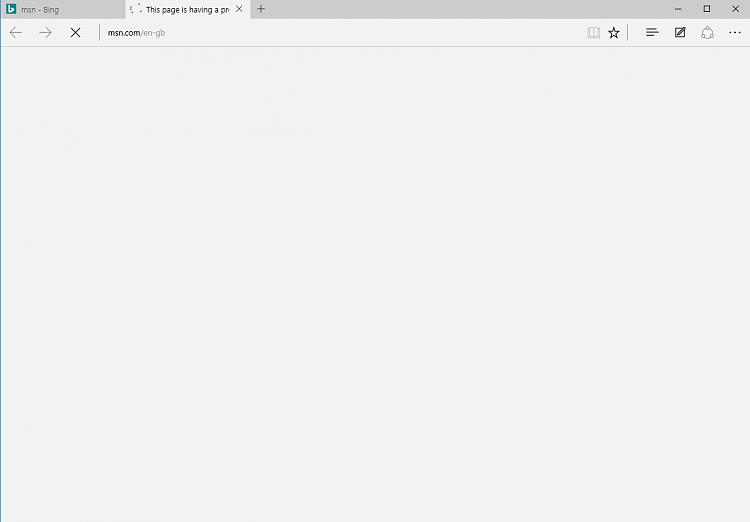In this image, a web browser window is displayed with a predominantly blank gray screen. In the top left corner, there are two tabs visible, and the second tab is selected, displaying a message that reads, "This page is having a problem." The uppermost part of the window features a gray bar where, on the top right, there are three icons: a minimized window icon, a maximized window icon, and a close window 'X' icon. Directly below this bar, the browser's address bar shows the URL msn.com. To the left of the URL bar, there are a backward arrow, a forward arrow, and a reload icon. To the right of the address bar, there is a star icon followed by four additional computer-related icons. The majority of the screen beneath these elements remains a light gray, blank background.